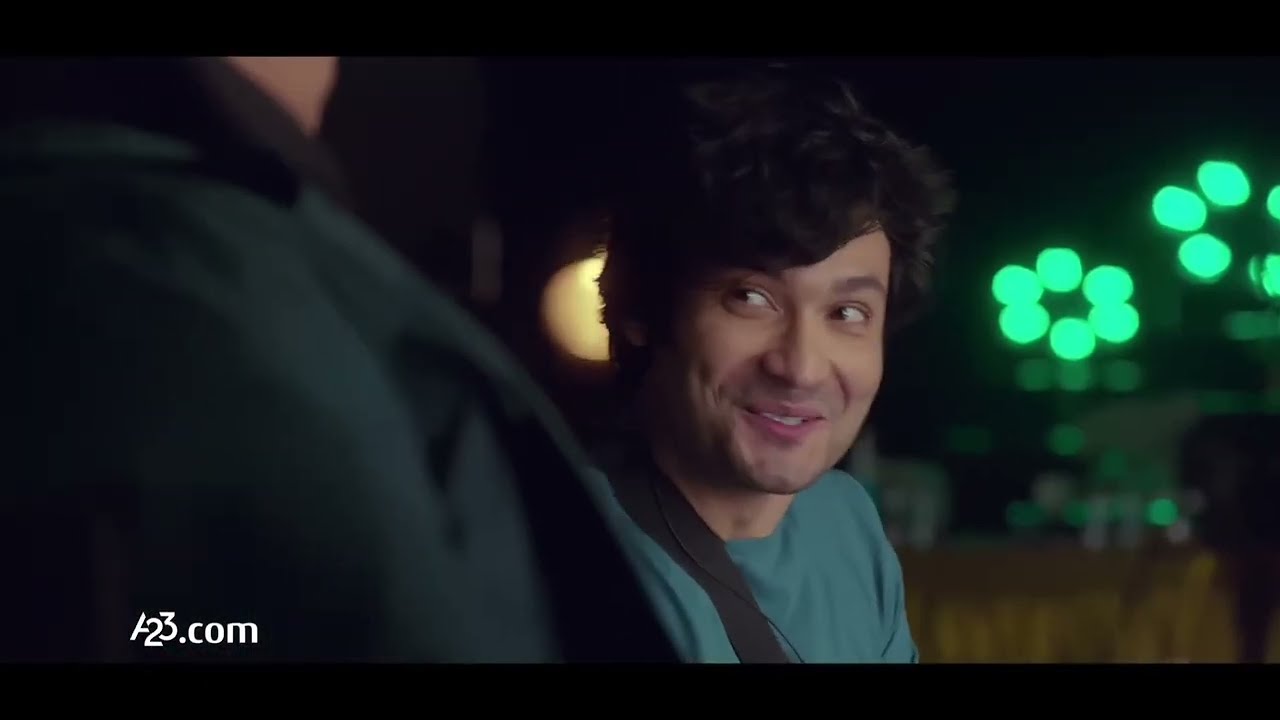This screenshot, presumably from a movie or video, captures a nighttime outdoor scene in a bustling city. A man with medium-length dark black hair is seen grinning or slightly laughing while looking to his left. He is dressed in a green t-shirt with a strap over his shoulder, suggesting he might be wearing a backpack. Another person, identifiable only by their green jacket with a black collar, is positioned in front of him; we can see their shoulder and the back of their neck. The background is blurred but illuminated by various lights, including a yellow circular light and some distinctive green lights arranged in a circular pattern. At the bottom left corner, there’s some white text that reads "a23.com." The image has horizontal black strips at the top and bottom, and the focus is primarily on the man's upbeat expression amidst the nighttime ambiance.